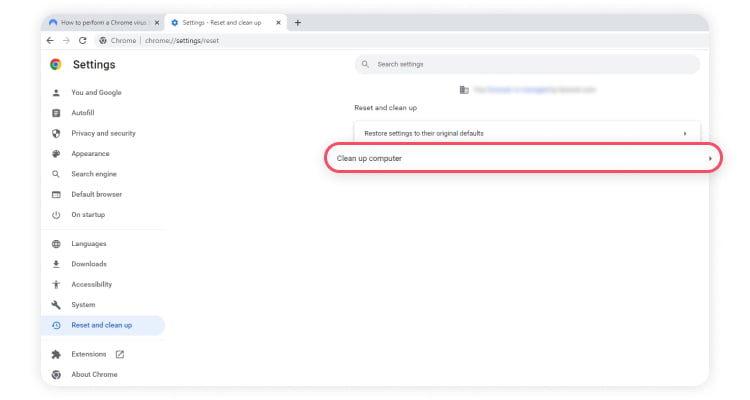The image captures a screenshot from a computer displaying two open tabs in a web browser, with the selected tab labeled "Settings: Reset and clean up." The active tab is identifiable by the text on it, indicating the reset and clean-up settings in Google Chrome. Below the tab title, the search bar reads "chrome://settings/reset."

On the left side of the screen, a vertical menu lists various settings categories, each accompanied by an icon symbolizing its function. The categories include "You and Google," "Autofill," "Privacy and security," "Appearance," "Search engine," "Default browser," "On startup," "Languages," "Downloads," "Accessibility," "System," "Reset and clean up," "Extensions," and "About Chrome." The "Reset and clean up" category is highlighted in blue, indicating it is selected.

To the right, against a white background, a light gray horizontal oval search bar at the top right corner displays the text "Search settings." Below the search bar, the text "Reset and clean up" appears in black. Underneath this, the option "Restore settings to their original defaults" is displayed, followed by a prominently outlined red horizontal oval containing the text "Clean up computer" in black.

The detailed layout and design elements clearly illustrate the Google Chrome settings interface, emphasizing the reset and clean-up options available to the user.